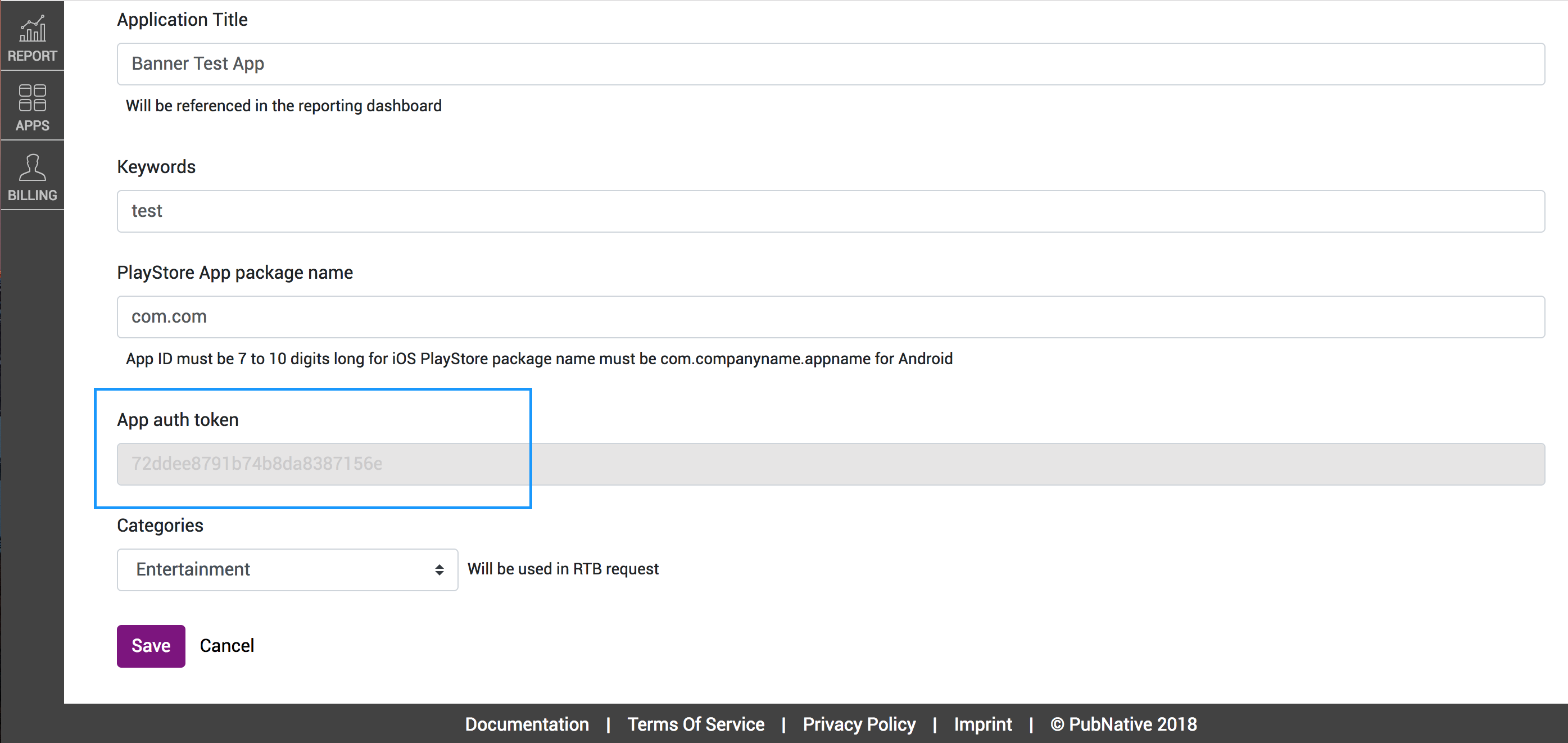On the left side, there is a vertical, thin rectangle with the headings "Report" at the top, followed by "Apps" and "Billing." 

To the right, there's a large white box. At the top-left corner of this box, there is a long search bar labeled "Application Title," with "Banner Test App" typed inside. Just beneath this, there's a reference to the reporting dashboard.

Further down, the word "Keywords" appears in bold black text, followed by another long informational box containing the word "test." Below this second box, "Play Store App Package Name" is displayed, with yet another long rectangle below it, containing "com.com." 

In smaller text beneath, there is an instruction: "App ID must be 7 to 10 digits long for iOS. Play Store package name must be com.companyname.appname for Android."

Next, inside a blue box, there is the label "App AUTH Token," followed by a gray rectangle with some very light text inside it.

Below this section, "Categories" is listed, and finally, in the lower-left corner, a purple square labeled "Save" is displayed, with "Cancel" to its right.